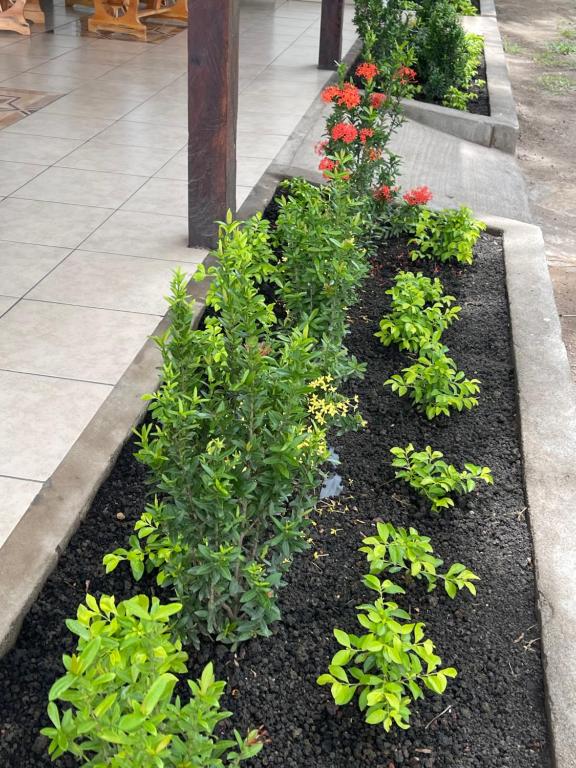This color photograph, taken in portrait orientation, features a detailed view of two planter beds set against a concrete backdrop, likely positioned outside a house near a kitchen area with cream and gray tiles. The scene captures a backyard or patio entrance, surrounded by several rectangular flower beds filled with dark, almost black planting soil. Each flower bed hosts rows of diverse green plants, with some taller shrubs placed at the back and shorter ones in the front. Among these plants, a flowering shrub with orange blooms stands out, while another smaller plant displays pink flowers. 

The image is framed by vertical wooden posts which appear on either side of a tiled ramp leading from a street to the walkway area. Furniture pieces like side tables and possibly a chair can be spotted in the background, along with support columns outlining the walkway between the flower beds. The surrounding yard has patches of grass interspersed with dirt, which could potentially become muddy when wet. Overall, the detailed composition of plants, tiles, and wooden structures creates a realistic depiction of a serene, well-maintained garden space.